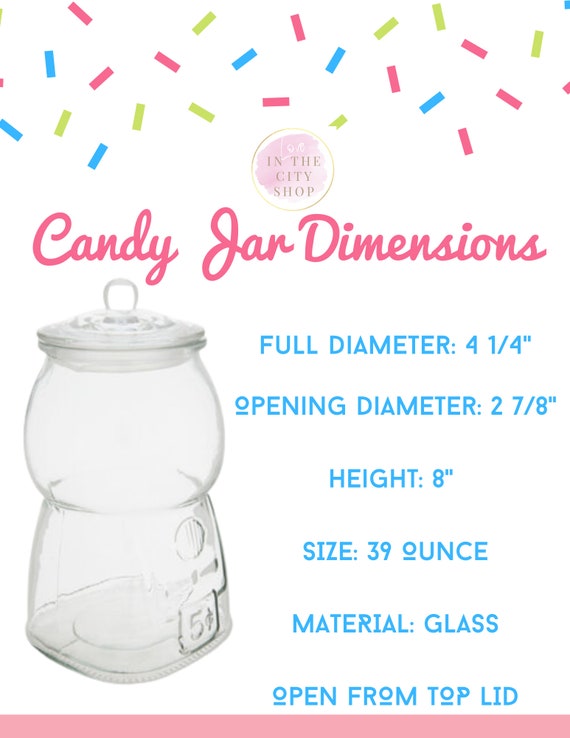This image displays the dimensions and features of a candy jar in a flyer-style layout. The background is white with festive confetti in red, blue, and green at the top. Just below the confetti is a circular insignia with a pinkish splash and brown text that reads "In the City Shop." The main title, "Candy Jar Dimensions," is prominently written in pink, cursive font. The central focus of the image is an illustration of a glass candy jar, reminiscent of an old-fashioned candy machine with a bulbous top, a narrow base, and a mechanism for inserting coins marked with "5 cents." To the right of the jar, the dimensions are meticulously detailed in light blue text: the diameter is 4 1⁄4 inches, the opening diameter is 2 7⁸ inches, the height is 8 inches, and it has a capacity of 39 ounces. The jar is made of glass and opens via a top lid. The bottom of the image is accented with a horizontal pink bar, adding a final touch of color to the flyer.